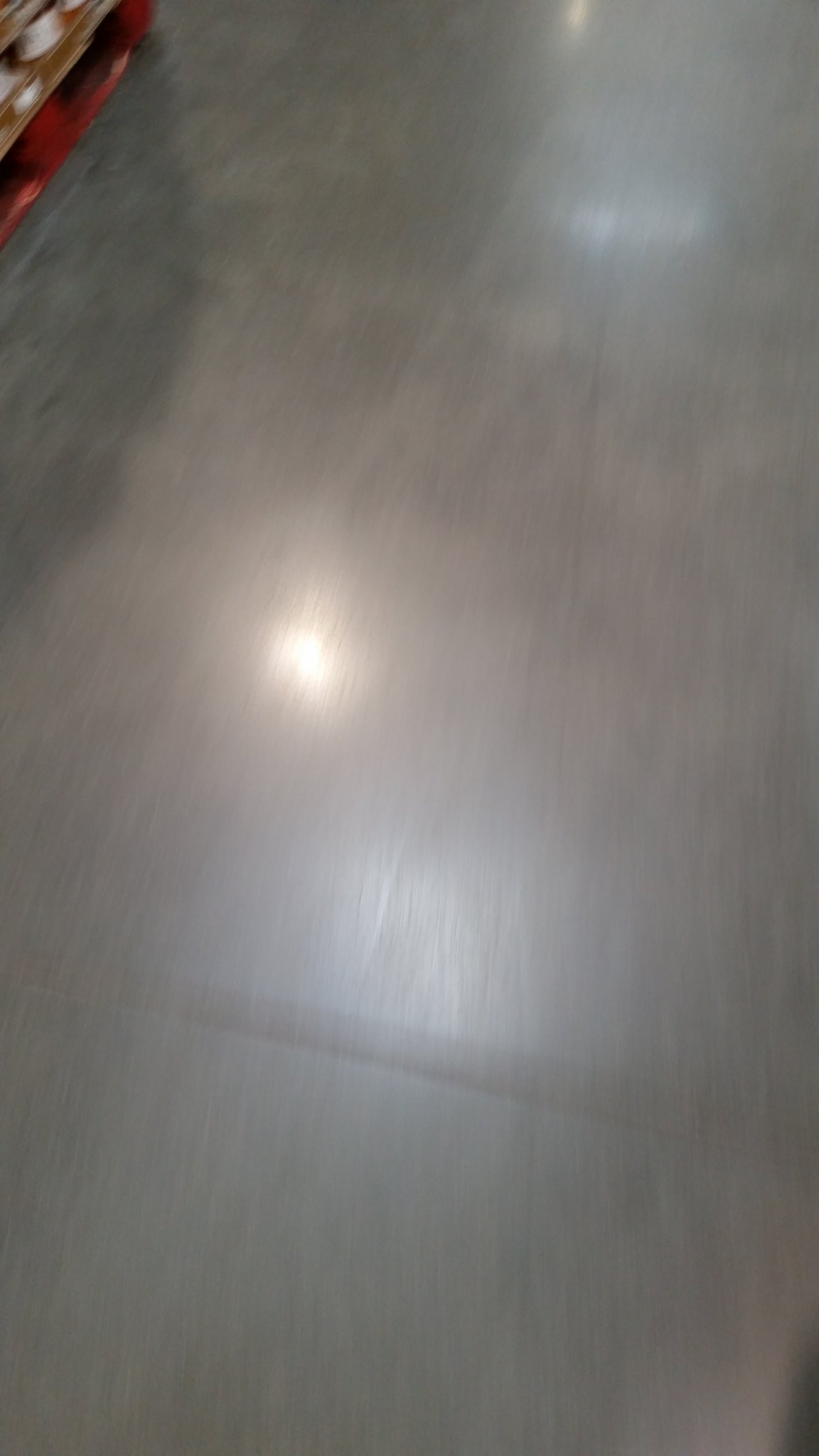This image depicts a somewhat blurry photograph of a shiny gray concrete floor, smooth as though it were a seamless sheet of linoleum, reflecting multiple lights from above. The primary light source is evident from a bright reflection on the right side and two additional, more diffuse reflections. In the upper left corner, there is a small visible section of a pallet-like brown and red object with a bit of white on top that casts a noticeable shadow to the left. The floor, although primarily gray, contains hints of brown and darker gray spots. On the bottom right, a dark spot contrasts with the overall shiny gray surface, further accentuating the reflective quality of the floor.